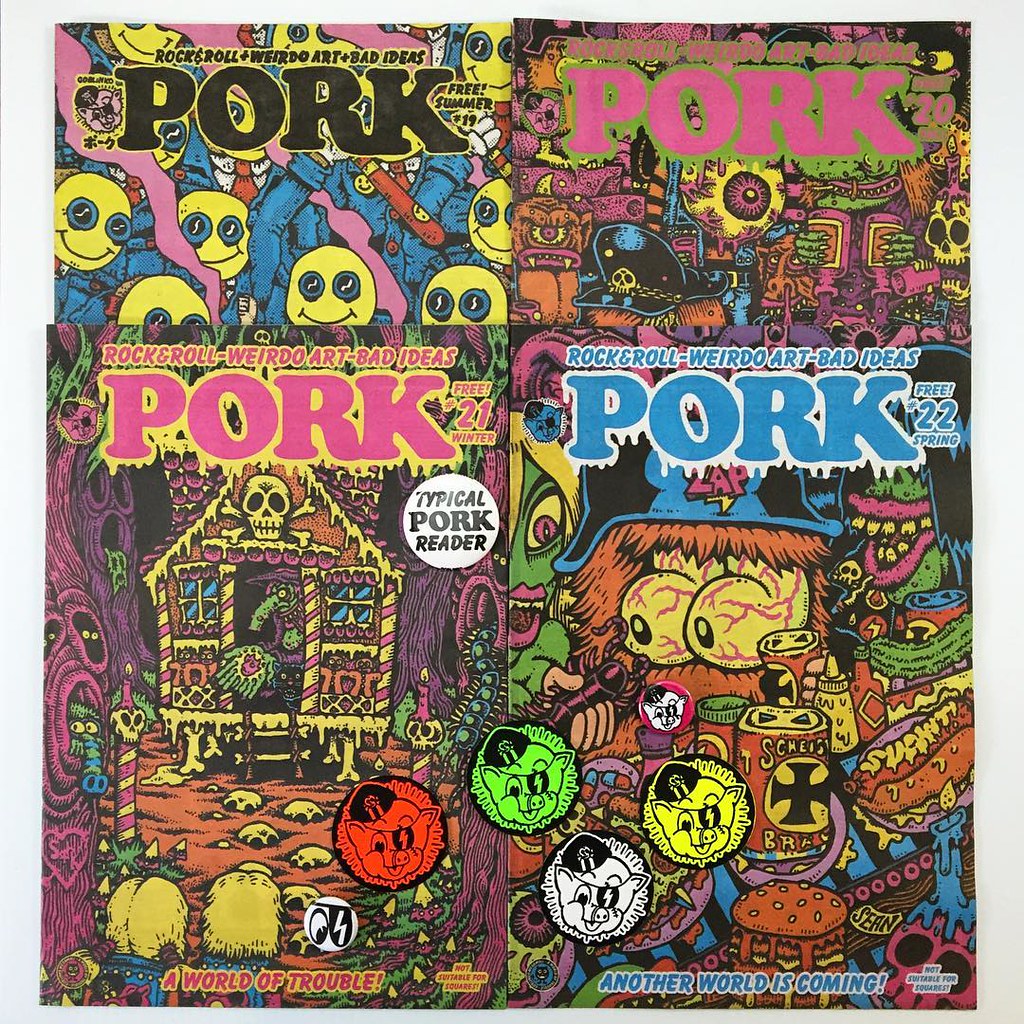The image showcases four vividly colorful comic book covers, emblazoned with the phrases "Rock-and-Roll Weirdo Art," "Bad Ideas," and prominently, "Pork." Each cover bursts with shades of bright pinks, blues, yellows, and greens, resembling glow-in-the-dark hues akin to late 60s or early 70s psychedelic style. The designs are richly detailed, featuring a house with skeleton head symbols, bone feet, an array of skeletons, skulls, worms, and pig faces in various colors—red, green, white, and yellow. The top left cover has black letters with a yellow border stating "for the summer of 19," while the top right has pink letters on a green background marked "summer 20." The bottom left reveals light pink letters with a bright yellow border noting "free 20, 21 winter," and the bottom right displays blue font with a white border saying "22 spring." Skeletons, crosses, eyeballs, and grotesque images frequent the designs, capturing an eerie yet vibrant aesthetic. The phrase "a world of trouble another world is coming" is inscribed at the bottom, encapsulating the chaotic and eclectic nature of the artwork.